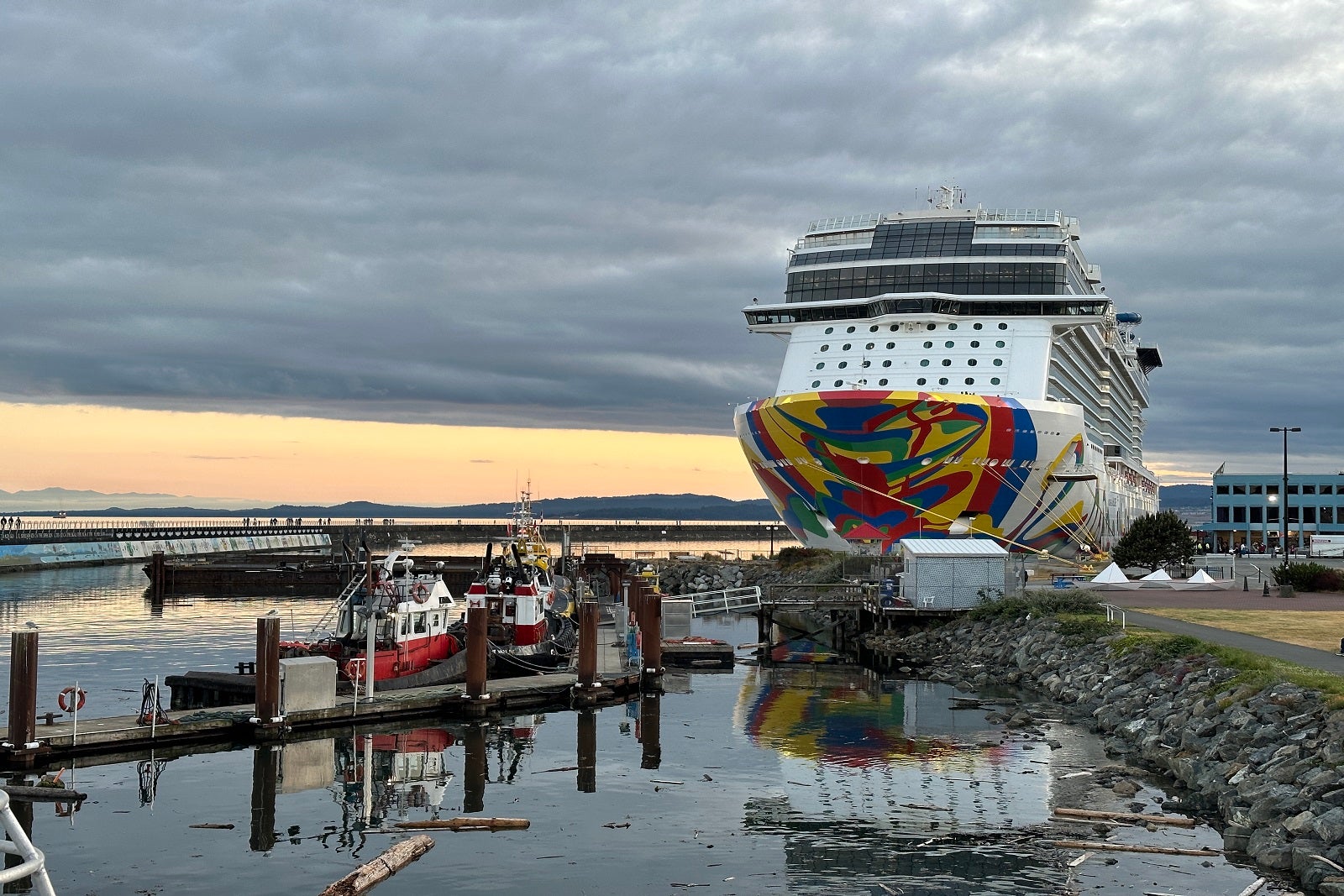The image captures a bustling cruise ship port during what appears to be either sunrise or sunset, evident from the golden and orange hues blending into a thick, gray, cloudy sky. Dominating the scene is a massive, multi-story white cruise ship with vibrant abstract designs in red, blue, yellow, and green painted on its front hull. The ship boasts about ten levels, with numerous windows along its sides and several stories at the top featuring clear glass windows. A notable feature is the large control deck situated about four stories from the top, equipped with panoramic viewing arms.

To the right of the ship, a multi-story building and surrounding parking lots are visible, suggesting activity and awaiting passengers. In the foreground, a smaller pier is lined with three or four tugboats, distinguished by their red, white, and yellow paint. The area showcases a rocky shoreline, both from the dock and stretching into the hilly distance. Floating chunks of wood add a touch of natural intricacy to the water by the pier.